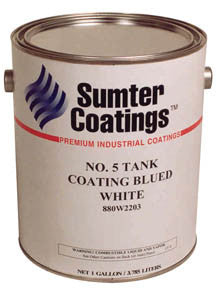The image depicts a standard paint can set against a white background. This can features a silver lid and a silver handle, currently positioned out of view, attached to its sides. The can's label is white and minimalistic, emblazoned with the brand name "Sumter Coatings™" in blue font. Below the brand name, in red font, the label reads "Premium Industrial Coatings." Further down, there are additional details in black font: "Number 5, Tank Coating, Blued White," followed by the product number "880-W-2203." The label also mentions the net volume of the can, "One Gallon" (approximately 3.7 liters). The can is slightly turned to the right in the image, allowing a view of metal knobs on the sides at the top. A small blue logo for Sumter Coatings is present as well. At the bottom of the can, a long black rectangle contains small black writing, providing additional product information.